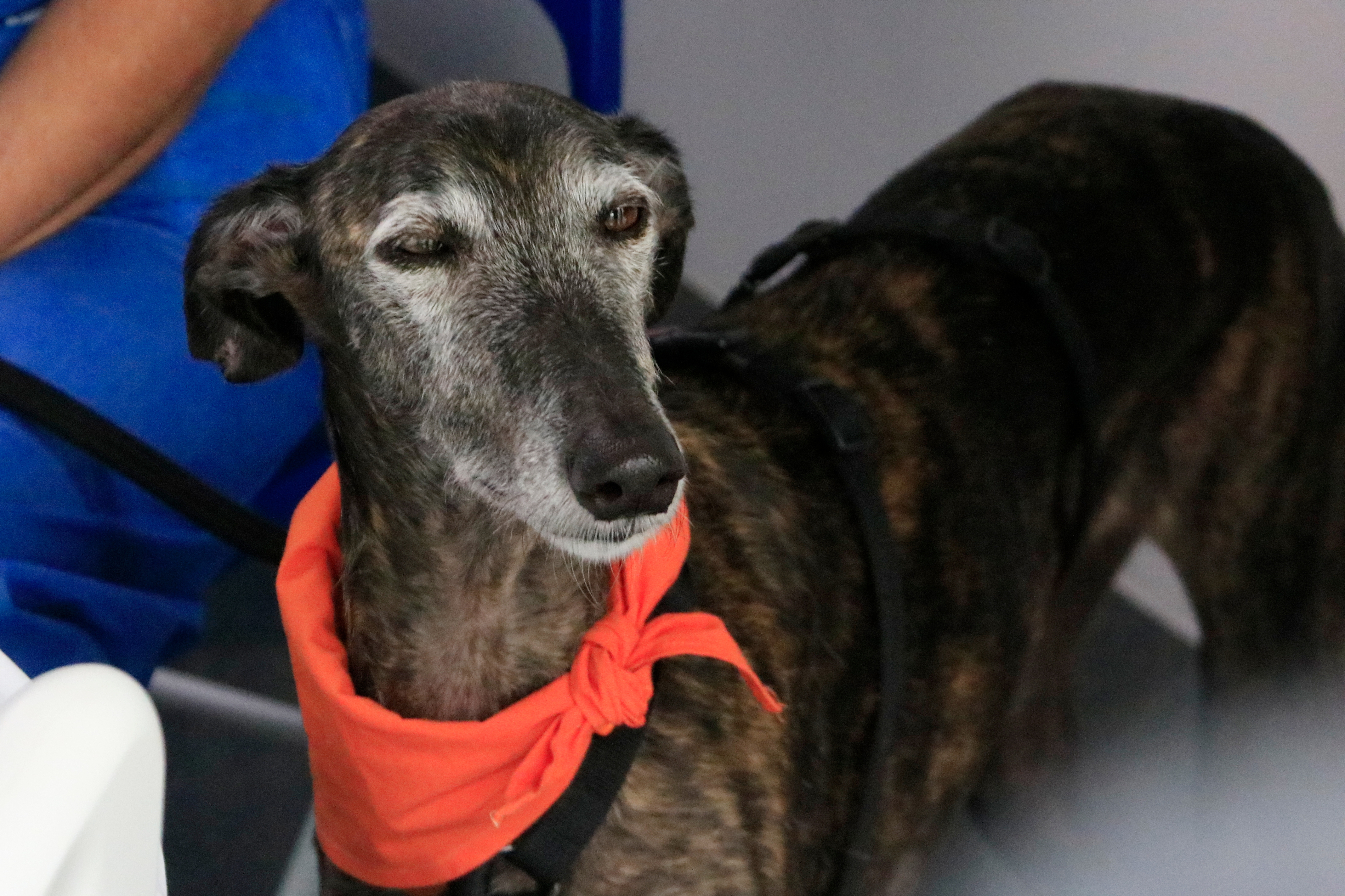In this rectangular photograph, which is longer horizontally than vertically, we see an elderly dog with a dark brown and black brindled coat; its face is marked by light gray fur around the eyes and nose, indicating its age. The dog's eyes appear cloudy, possibly due to cataracts, and its ears are laid back. It has a long neck adorned with a bright neon orange bandana tied loosely, beneath which a black harness or collar is faintly visible. The dog’s nose is black, and its eyes are slightly squinted as if reacting to a light source. Only the dog's body and head are visible; its feet are not shown.

Next to the dog, there is a person seated in a blue chair, partially visible, wearing a blue dress. Only the person's arm and a part of their pants are clearly seen, with the arm appearing in the upper left corner. The person might be holding a black leash that is attached to the dog, though the leash is behind the dog and not clearly visible. The ground in the image is gray, and the backdrop features a white wall. Additionally, there is a piece of white plastic in the lower left corner, possibly a part of the chair. The overall scene suggests this may be a service or support dog.